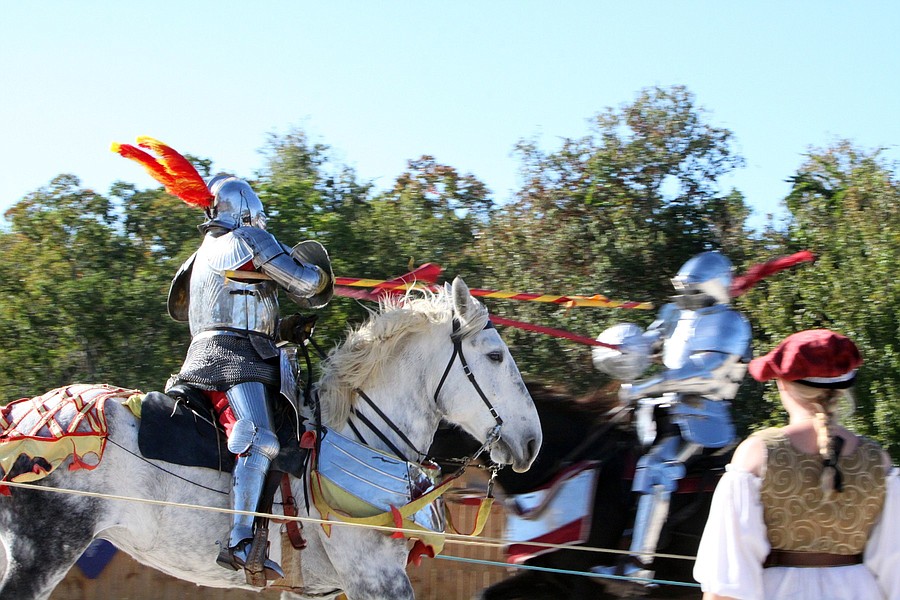This image, likely taken at a Renaissance Fair or a similar reenactment event, depicts a dramatic jousting scene. Two fully armored knights are engaged in combat on horseback under a bright blue sky with lush green trees in the background. On the left side, a knight on a striking white horse is prominently in focus. The horse's tack is adorned with a shiny chrome collar and vibrant red and yellow fabric, with a detailed blanket draped over its back. The knight wears gleaming silver armor with a chainmail skirt, topped with an extravagant helmet embellished with large red and yellow feathers. He grips a matching red and yellow striped lance, poised for action. 

Opposite him, to the right, is another knight on a black horse, slightly out of focus. This knight holds a red lance, and his horse is equally striking. In the foreground, a spectator is visible from behind. She wears a distinctive red hat with her blonde hair styled in a braid tied with a black bow. Her outfit includes a brown brocade vest over a white blouse with flowing sleeves, and a white skirt. The scene is framed with a yellow rope running along the bottom, marking the boundary of the jousting arena.